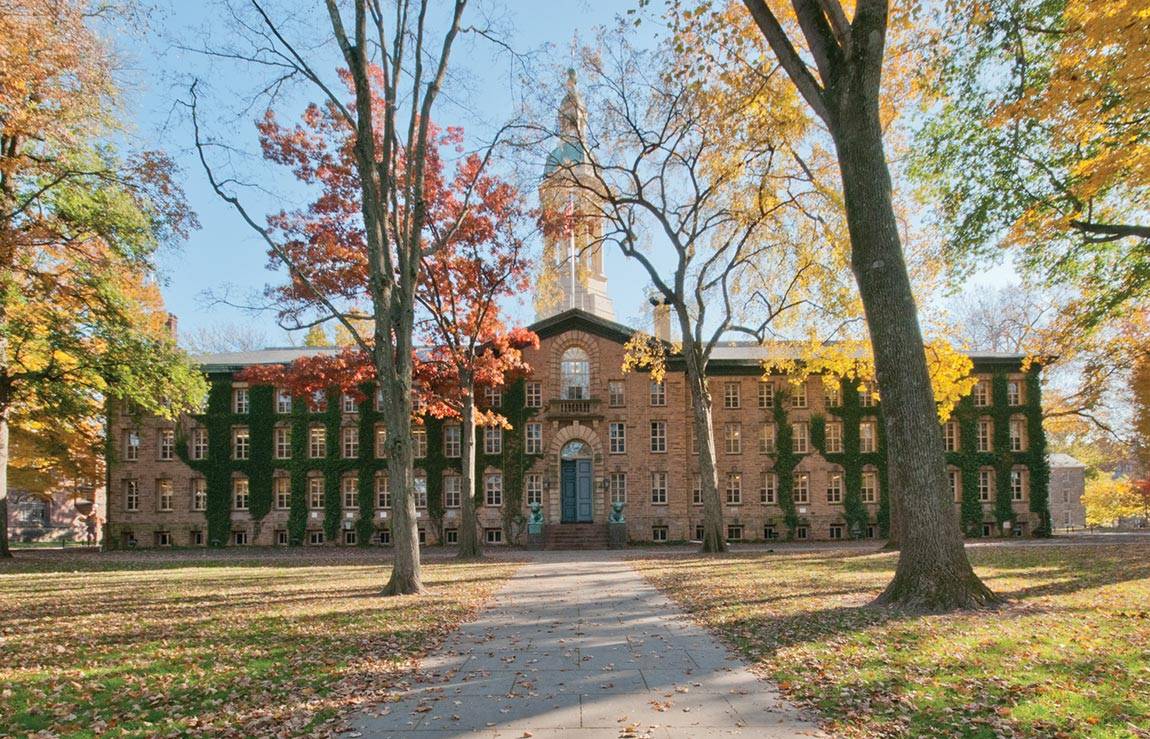This image captures an impressive, old building that resembles a university or college campus. The structure is rectangular and spans four stories, with a defining steeple or copula at the top, featuring a green tip. The light brick facade is interspersed with patches of green ivy or moss, especially around the evenly spaced windows. The central portion above the two front doors showcases a distinctive palladium window and a small porch area. Flanking the entrance are two gargoyles. Leading up to the building, there's a wide concrete sidewalk that is bordered by large trees in various stages of autumn transformation, adorned with vibrant reds, yellows, oranges, and some green leaves. The trees, partially bare, suggest a quintessential fall scene, especially as the sun illuminates the scene from the right-hand side, enhancing the seasonal colors and the aged elegance of the building.